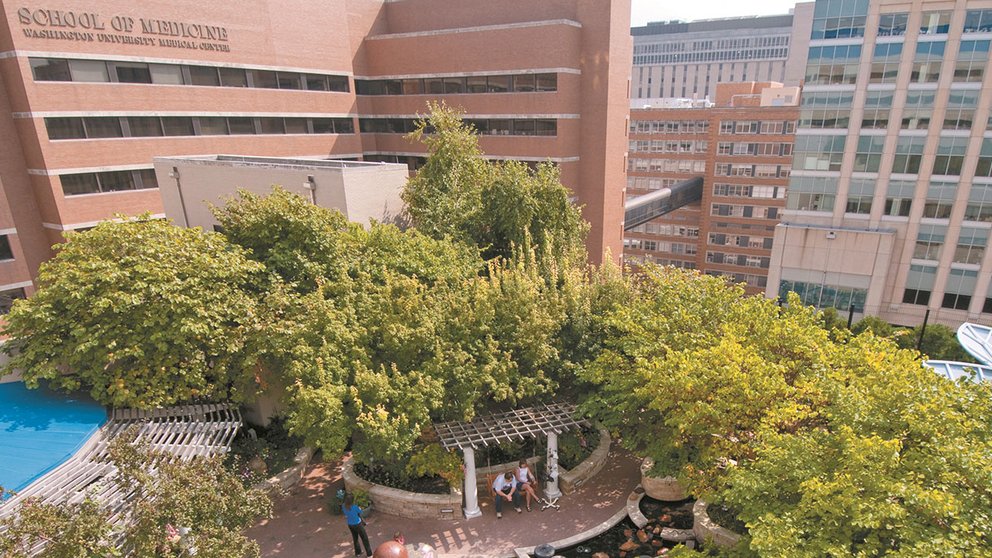The image captures a bright, clear, drone's-eye view of Washington University Medical Center's School of Medicine. Dominating the left side of the image is a large, reddish-orange, L-shaped building labeled "School of Medicine, Washington University Medical Center," which features several stories and black rows of windows. This main structure connects via an elevated catwalk to another nearby building. Below, the scene narrows into a vibrant courtyard surrounded by lush deciduous trees, indicating spring or summer. The courtyard features a shaded trellis area with a bench where a man and a woman are seated, while another woman stands nearby. Scattered throughout are white planters, circular pots, and white fencing, adding structured greenery. To the left, an ambiguous blue element might be a pool or a tarp. Beyond the campus area, several high-rise buildings form the city's skyline, accentuating the medical center's urban setting.